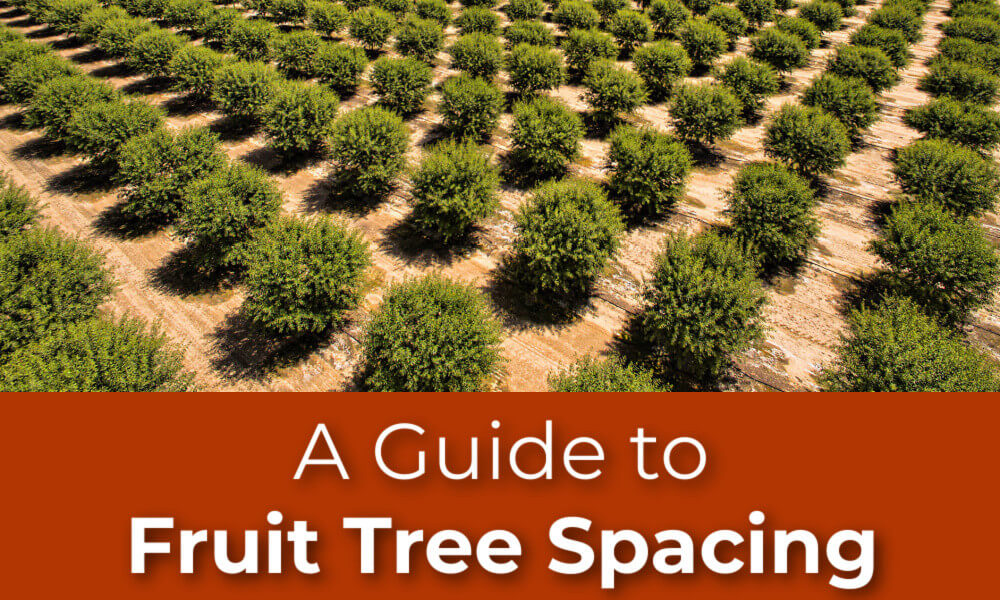This aerial photograph showcases an expansive orchard with neatly organized rows of green, bushy trees. The trees are evenly spaced, with light brown dirt visible in the gaps between the rows. The sunlight, coming from the upper right corner, casts shadows of the trees towards the lower left, creating a darker hue on the ground in the shaded areas. At the bottom of the image, a dark red banner is prominently displayed, with white text in two lines. The top line, in thinner block letters, reads "A GUIDE TO," while the second line, in larger, bold block letters, declares "FRUIT TREE SPACING." The meticulous arrangement of the trees and the informative banner contribute to a comprehensive visual guide on orchard spacing.